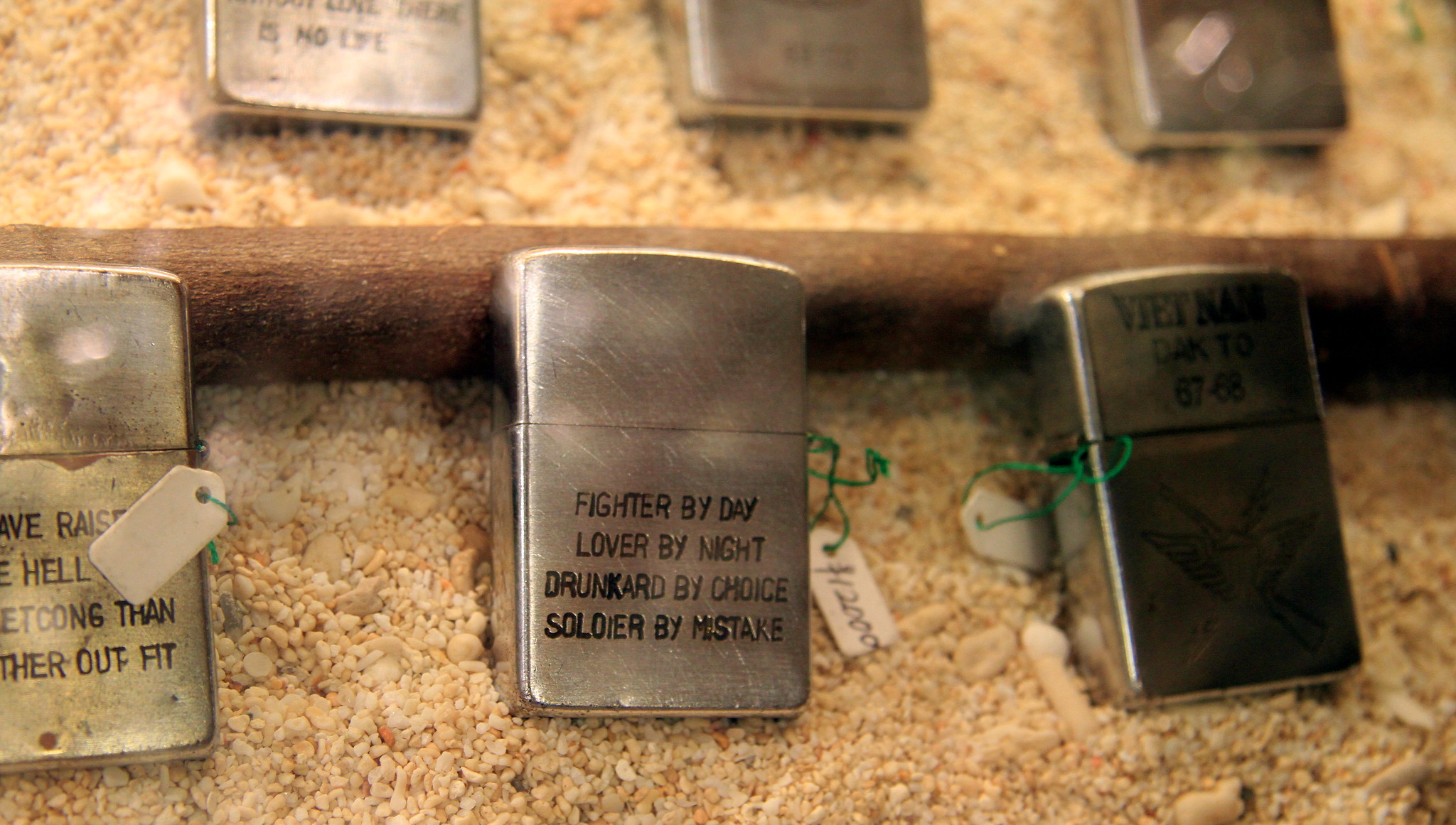This horizontally aligned rectangular photograph captures a display of six silver, rectangular Zippo lighters. These lighters, with a vintage appearance, are arranged in two rows of three, set against a background of fine beige and white rock fragments. The top row of lighters is slightly blurred. In the center of the bottom row, a prominent lighter displays the inscription "Fighter by day, lover by night, drunkard by choice, soldier by mistake" in black print. It has a small white price tag attached with a green string, marked "12000." To its right, another lighter bears the text "Vietnam DAC 267-68" alongside a blurry symbol, also tagged similarly. The lighter on the left side appears worn and has text that is partially cut off by the edge of the photograph. All lighters are affixed with green-threaded price tags, indicating they might be for sale, possibly at a flea market. The lighters are propped up by a wooden platform, enhancing their display against the sandy gravel-like backdrop.